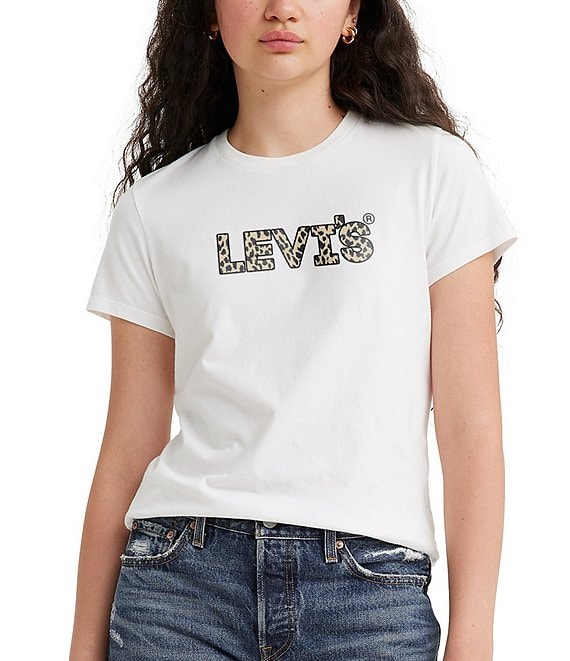The image is a professional, full-color photograph of a young woman, likely in her 20s, set against a stark white background. She is depicted from just below her nose to about her hips. The woman has long, curly dark brown hair that cascades down to about her shoulder blades and is adorned with hoop earrings. Her facial features include a small nose and fairly full lips. She is wearing a white, short-sleeved Levi's t-shirt, which prominently displays the brand's name in a cheetah print pattern along with the registered trademark symbol. Below the shirt, she is dressed in blue jeans that appear slightly distressed with a small rip above the pockets. The jeans have a button at the top and pockets on both sides, likely also a Levi's product. No additional jewelry is visible in the image.